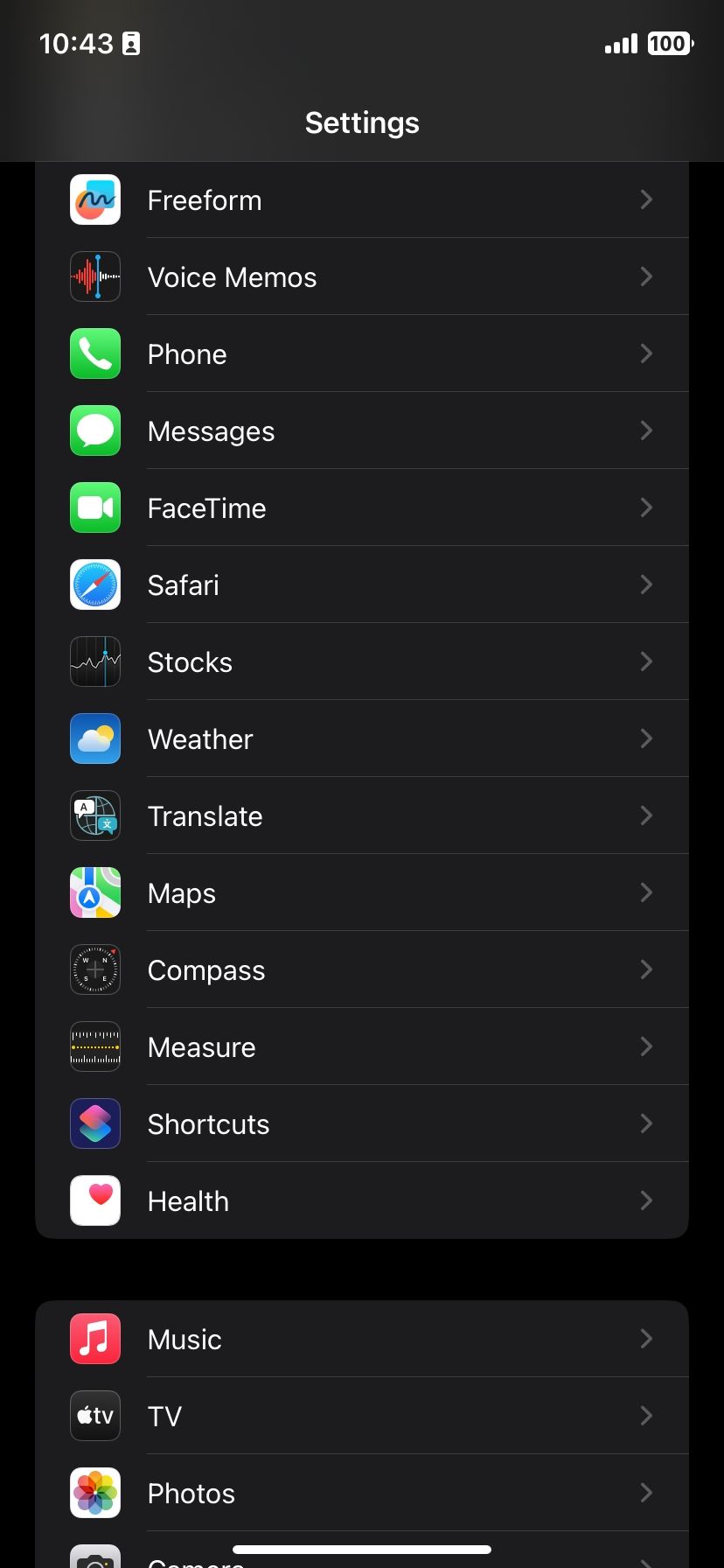This is a vertical rectangular screenshot from a smartphone, featuring a predominantly black background. At the top of the screen, in white text, the time is displayed as "10:43" followed by a user icon. In the top right corner, the status indicators show a full four bars of signal and a 100% battery level. The central portion of the image is dominated by the word "Settings" in a larger white font. Below this, there is a comprehensive list of installed apps presented in a vertical arrangement. The first section includes the apps: Freeform, Voice Memos, Phone, Messages, FaceTime, Safari, Stocks, Weather, Translate, Maps, Compass, Measure, Shortcuts, and Help. After a small gap, the list resumes with the apps: Music, TV, Photos, and Camera, concluding the visible inventory of applications.